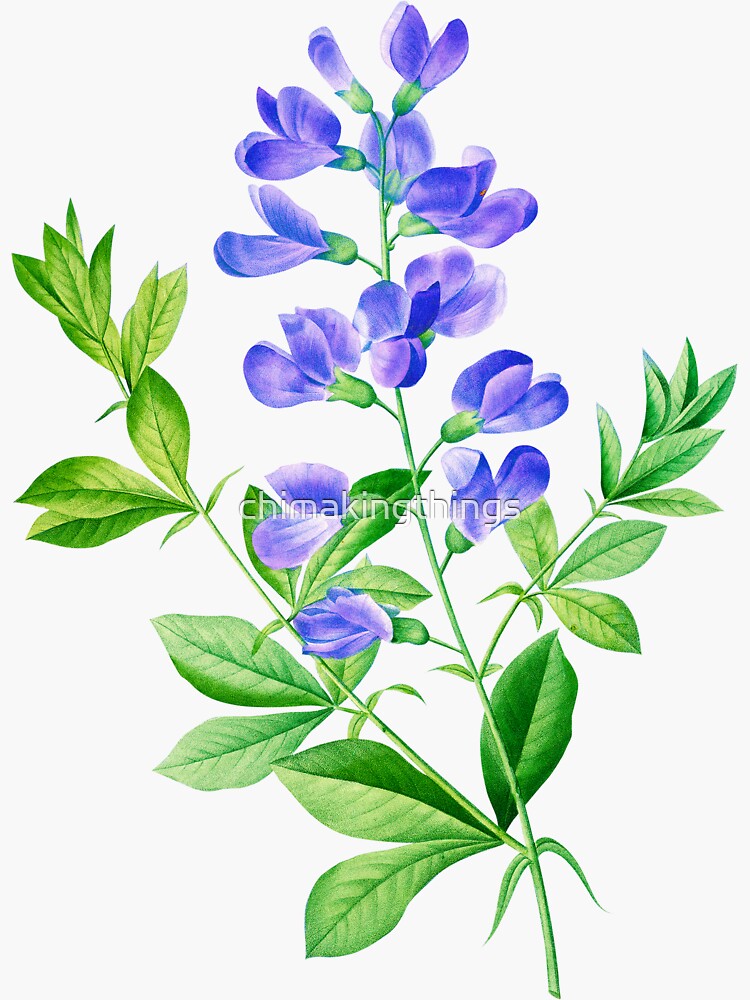The image depicts a detailed botanical illustration of a delicate, vibrant purple flower with blue undertones, set against a light gray background. The rectangular composition is oriented in a portrait format, with the height twice the length of the width. The primary subject is a central thin green stem, which extends vertically and culminates in multiple green buds at the top. From these buds, the petals fan out gracefully, much like butterfly wings, in shades of purple and blue. Each flower, displaying between two to four petals, is attached to a green, bell-shaped cap under the bloom. Midway down the main stem, two smaller branches extend outward, adorned with almond-shaped leaves that feature distinct dark green veins. The bottom of the central stem is cut off toward the bottom right of the image. Across the entire illustration, there is a semi-transparent white text watermark reading "SHIMA KING THINGS," lending a subtle overlay. The artwork is a striking representation of botanical elegance, capturing the flower's fresh, vibrant, and delicate beauty.